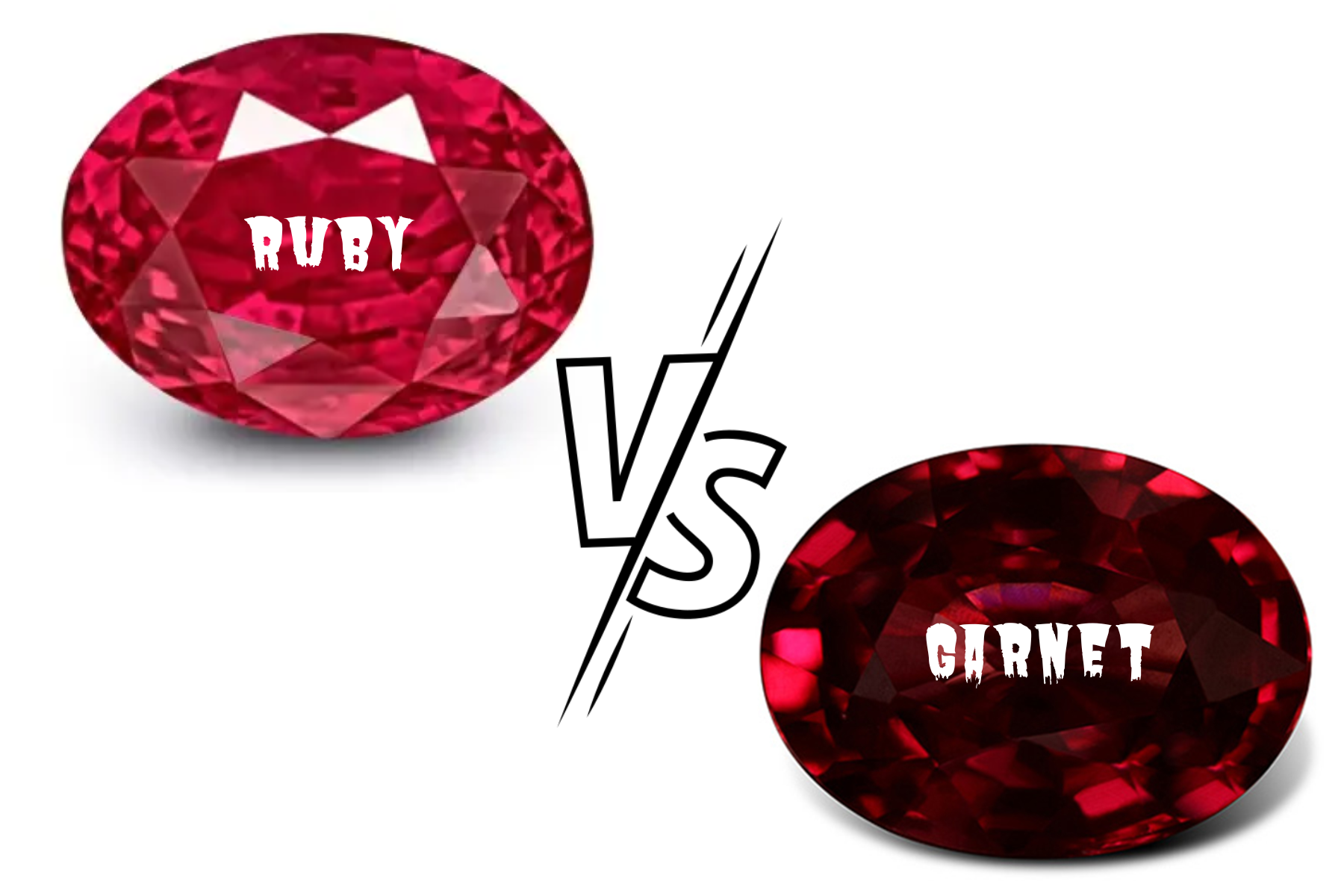This is a detailed color photograph featuring a comparison between two gemstones: a ruby and a garnet, set against a white background. On the upper left corner is an oval-shaped, bright red, almost transparent ruby with white text lettering "RUBY" in all black letters and two arrows pointing upward. The lower right corner showcases an oval-shaped, dark red, slightly transparent garnet with yellow capital letters spelling "GARNET." In the center of the image, there is a bold "VS" in black text with a white center, indicating the comparison between the two gemstones. The photograph appears to be shot directly from above, emphasizing the vivid colors and details of both stones, with the digitally imposed text complementing the composition.